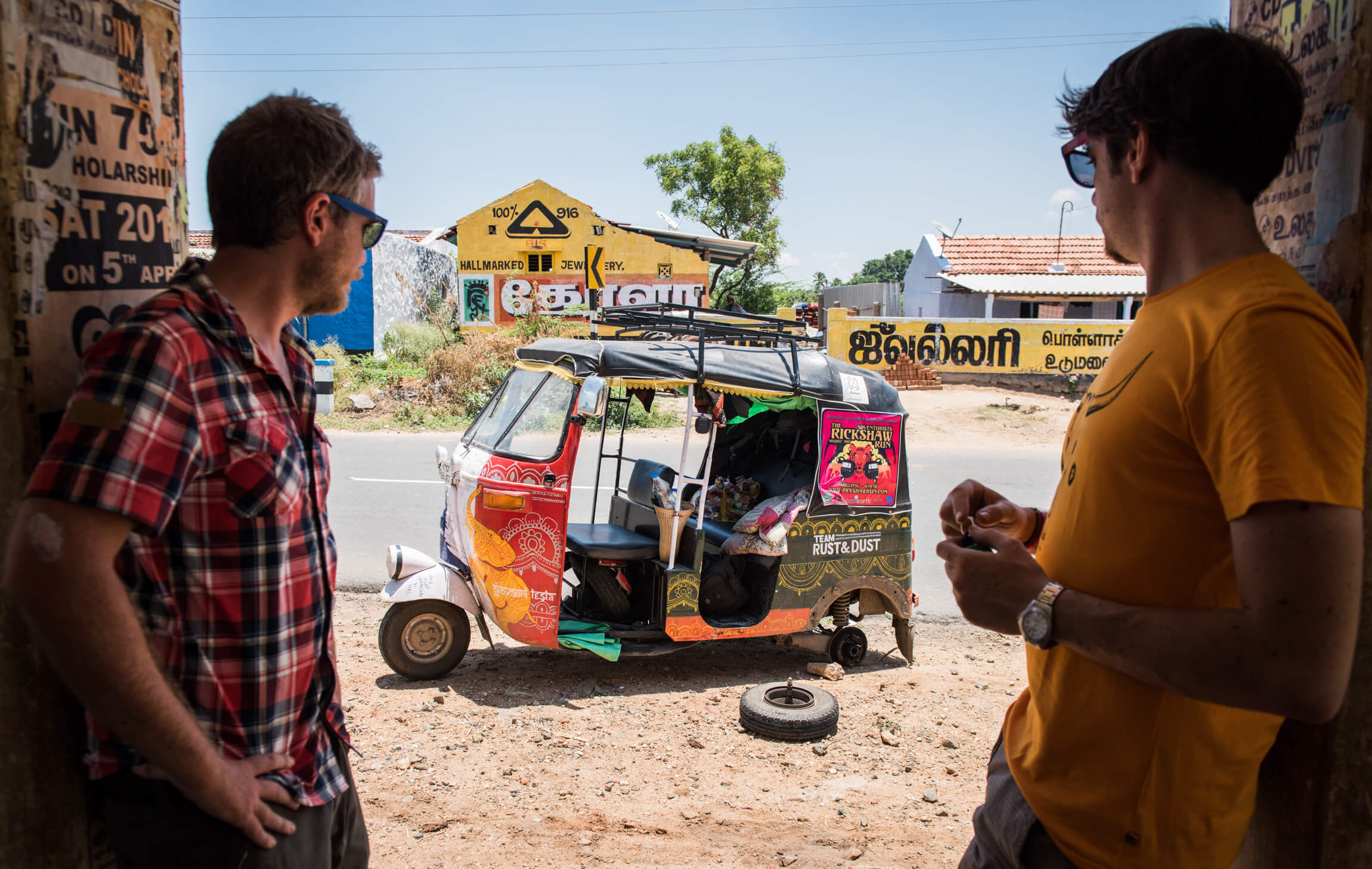In this captivating photo, two men—one of Caucasian descent wearing a red shirt, and the other of Indian descent in a yellow shirt—stand on either side of a large, open doorway. Both are wearing sunglasses and appear to be in a desolate, dry place, possibly a desert. They are intently staring at a colorful, cart-like vehicle resembling a rickshaw or golf cart. The vehicle, labeled "Rust and Dust," features posters and a small black roof cover but seems to be in disrepair with one of its wheels detached, lying on the gravelly dirt road.

In the background, a mix of under-construction buildings and structures adorned with graffiti and yellow tape marked with a foreign language are visible, further framing the vibrant yet somewhat rundown scene. Above, the blue sky stretches out with sporadic trees providing a touch of greenery to the arid landscape. The two men’s serious expressions and the vehicle’s condition suggest they might be contemplating how to repair it.